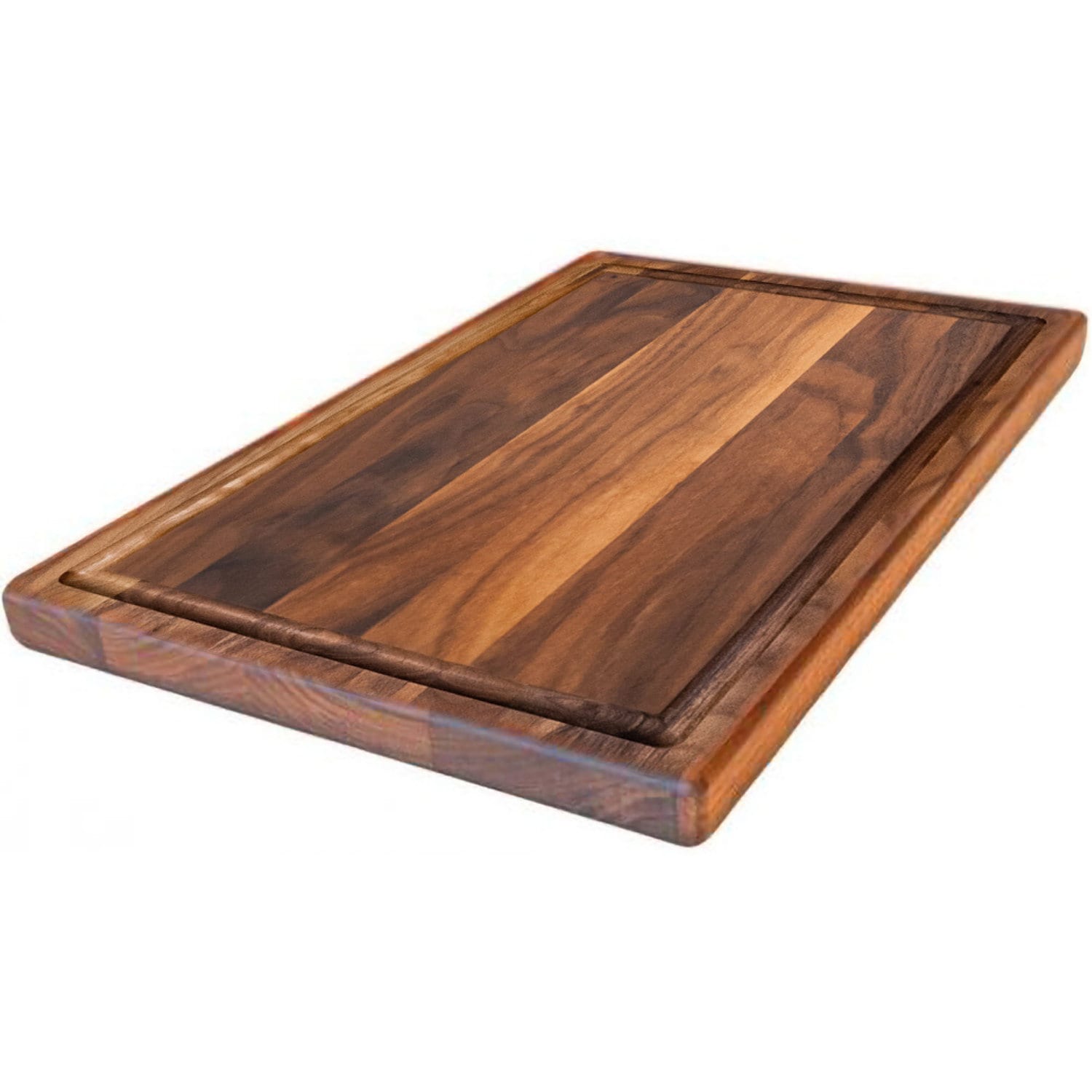This image features a pristine, rectangular wooden cutting board, expertly displayed at a diagonal angle against a white or possibly transparent background. The board showcases a striking contrast in wood stain, with the central panel appearing lighter than the darker-stained edges, highlighting the natural wood grain throughout. A prominent feature of the board is a deep groove running close to its perimeter, approximately one centimeter in from the edge, typical of high-quality cheese boards or trays. The board's clean and untouched appearance suggests it may be a new or display model, ideal for marketing purposes or an online catalog, presenting it as an elegant and functional kitchen accessory.